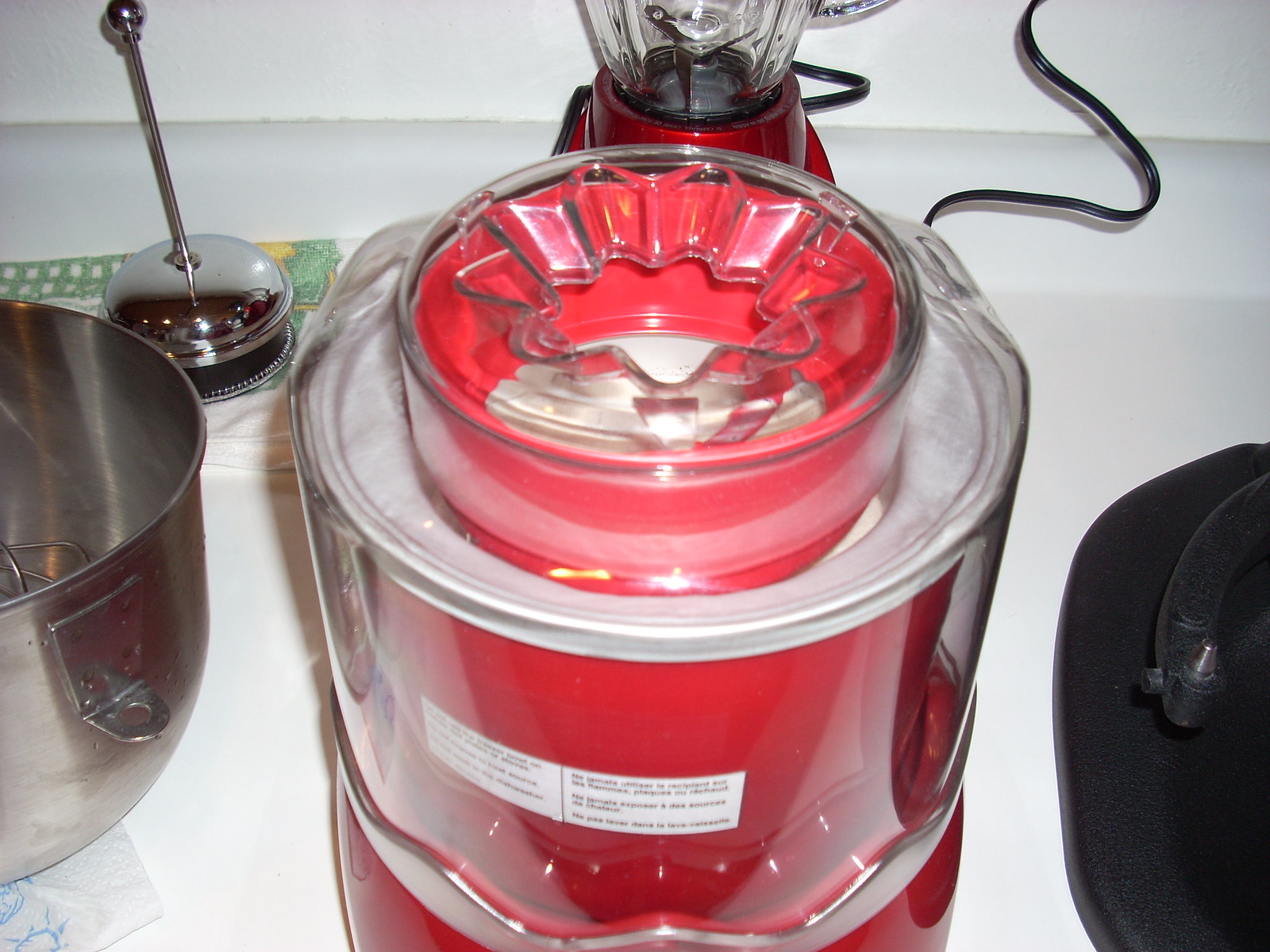This color photograph displays an assortment of kitchen appliances set against a pristine white background. Dominating the center of the image is an intriguing red kitchen device with a transparent glass cover, adorned with white labels featuring illegible black text. The device includes an irregularly-shaped opening at the top, resembling a floral pattern, and is connected to a black cord extending toward the top right of the frame.

To the left of this central appliance, a stainless steel pot with a handle featuring a small hole is placed atop a white tissue, partially decorated with a blue design. Inside the pot are silver wires and a silver substance. Additionally, a white cloth with green and yellow designs lies beneath the pot, contributing to the intricate detailing of this setup.

Further left, the photo reveals a steel bowl, potentially part of a kitchen aid or mixer attachment. Above this bowl sits the top part of a silver French press for coffee. At the far right of the image, partially cropped out, a black appliance appears, characterized by a black handle with a silver tip.

In the uppermost section of the image, a familiar kitchen appliance—a blender—rests. Its design includes a glass pitcher with a red base, a visible internal blade, and a black cable extending outward. The cohesive arrangement of these appliances, enhanced by their contrasting colors and materials, creates an engaging and detailed kitchen scene.